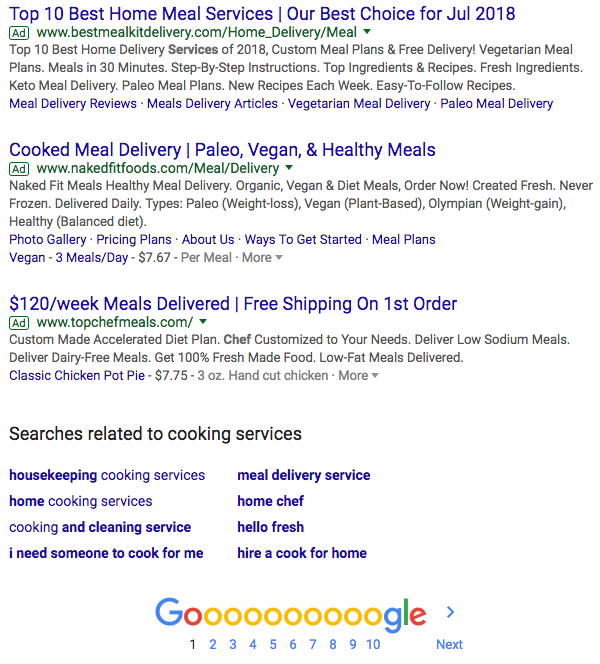**Caption:**

At the top of the image, bold blue text reads, "Top 10 Best Home Meal Services," followed by a thin vertical line and the phrase, "Our Best Choice for July 2018." Below this heading, enclosed within a green square, is the word "Add" next to a clickable link: www.bestmealkitdelivery.com-homedeliverymeal. 

The next section features a blue heading: "Cooked Meal Delivery - Paleo, Vegan, and Healthy Meals," accompanied by another green box containing the word "Add" and a link: www.nakedfitfoods.com-meal-delivery. 

Further down, the image displays "$120 a week, Meals Delivered," followed by a vertical line and the offer "Free shipping on first order." Below this offer, there is a small green box with the link: www.topchefmeals.com.

Continuing downward, the image lists "Searches Related to Cooking Services" in bold blue text. The related searches include:
- Housekeeping Cooking Services
- Home Cooking Services
- Cooking and Cleaning Service
- I Need Someone to Cook for Me
- Meal Delivery Service
- Home Chef
- HelloFresh
- Hire a Cook for Home

At the very bottom, the word "Google" appears with an exaggerated series of yellow "O"s, prominently standing out.